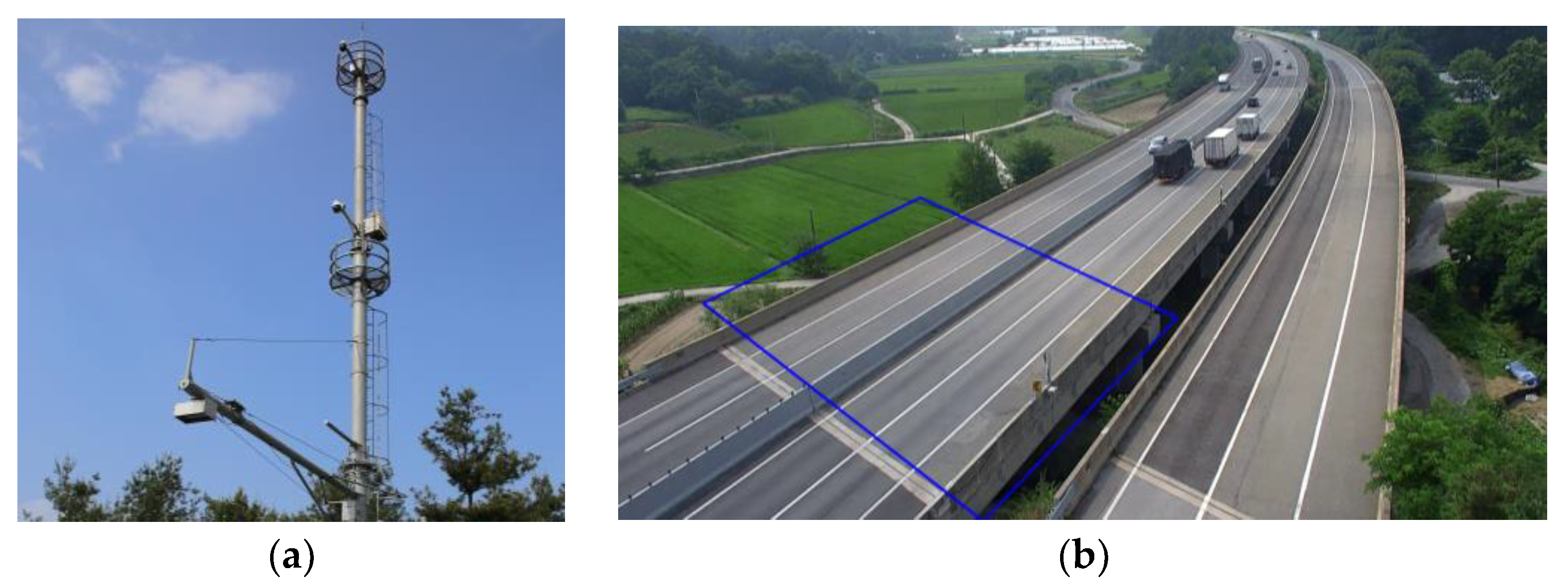The image is composed of two separate snapshot photographs arranged horizontally, labeled beneath each as (A) and (B). The left photograph (A) features a metal electrical tower set against a blue sky with scattered white clouds. The tower has three round lookout areas, a ladder on the side, and an extending metal arm resembling a street light. Visible below the tower are tree tops. This photograph has a snapshot quality and lacks professional polish.

The right photograph (B) provides an aerial view of a freeway with three lanes, curving from the bottom-left towards the top-right. The highway is accompanied by green fields, trees, and smaller roads. The scene includes a few trucks and other vehicles scattered across the lanes. A specific section of the freeway is highlighted with a blue overlaying text box. This image gives a broad, detailed perspective of the road and surrounding landscape, contributing to the overall composition, which appears to be suited for a textbook or educational material.